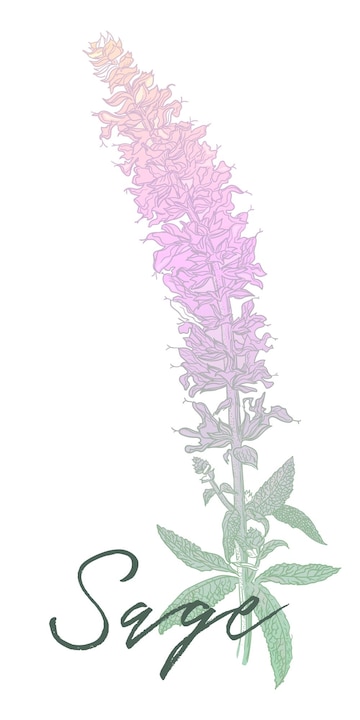The image is a detailed, botanical-style color illustration of a sage plant against a white background. The plant features a long, slightly arcing stem with a dense cluster of tubular flowers extending throughout. The stem starts at the base with a few pale green, textured, and curly leaves that exhibit numerous veins. The flowers transition in a gradient from a pale pinkish-purple with a slight peach tint toward the top of the blossoms. At the bottom of the image, the word "sage" is written in a hand-painted cursive font, colored in red with a natural, handwritten style. The overall composition is in portrait orientation, providing an elegant and detailed study of the sage plant.